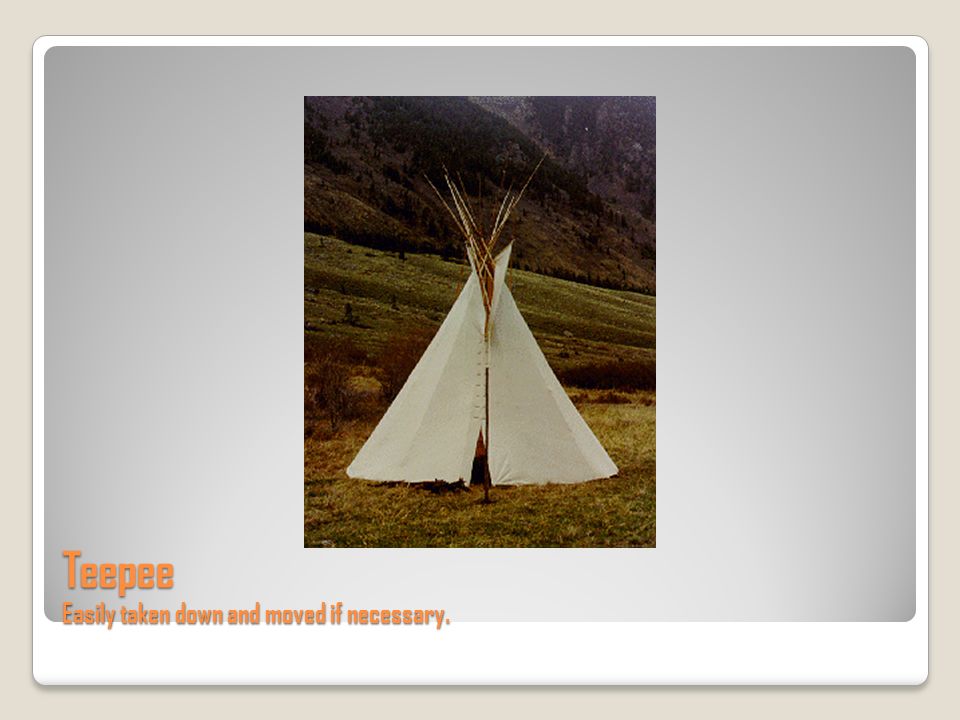The image showcases a traditional white teepee made of fabric supported by natural, whitish sticks protruding from the top. The teepee has visible buttons and a slight crease in the middle, and stands on a patch of mostly brownish, somewhat dry grass with greenish areas nearby. In the background, there is a landscape featuring trees and a large hill or mountain with vegetation, some parts of which appear to be bare dirt. The image is set against a light gray background, enclosed by a white round border, and framed again by a light gray beige flat background. At the bottom left of this framed area, in light orange lettering, it prominently states "teepee" with a description beneath reading "easily taken down and moved if necessary."